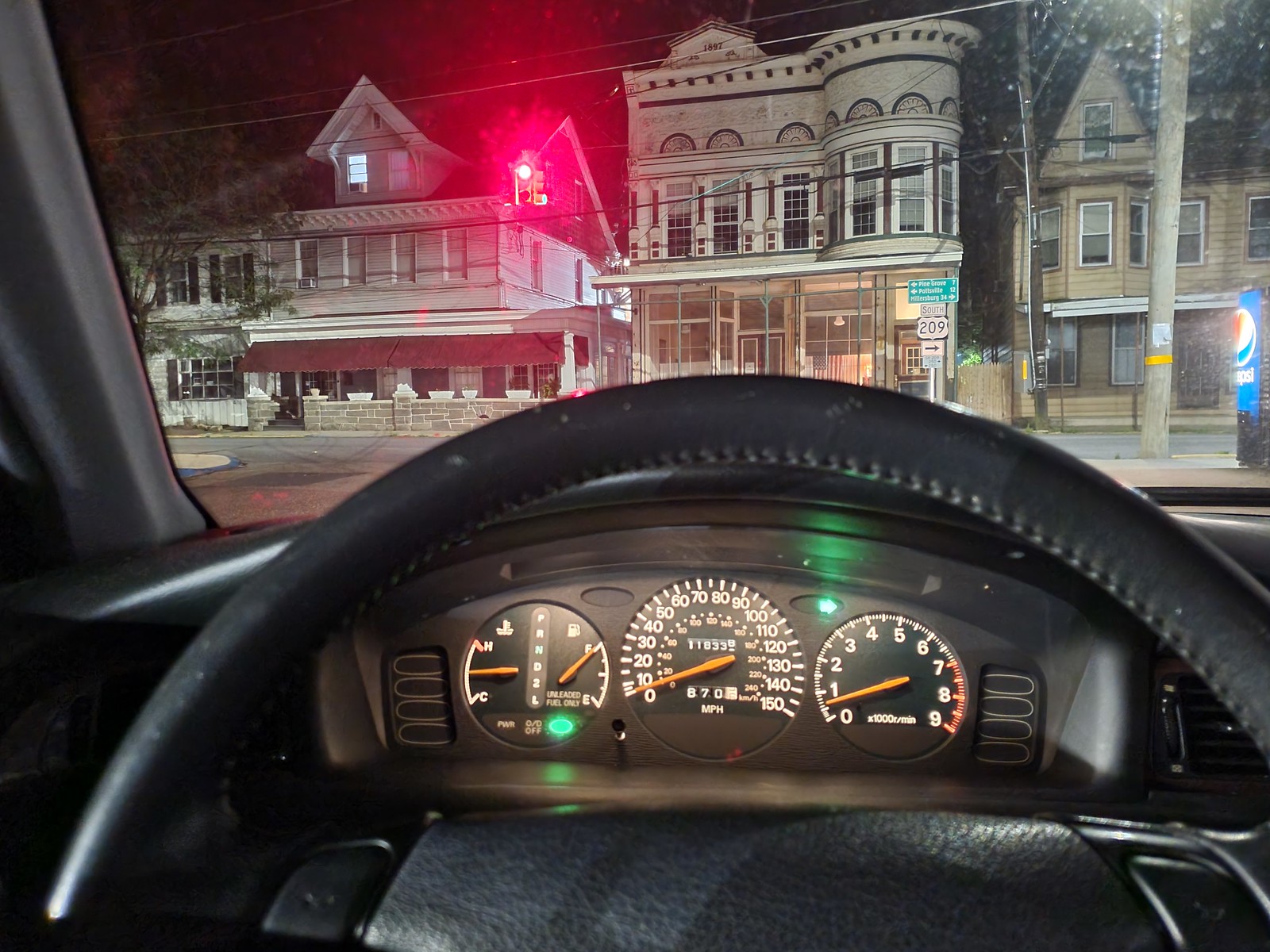This nighttime photograph captures a view from inside a parked car, looking out onto what appears to be a charming city street. Dominating the foreground is a large, black leather steering wheel, accompanied by a detailed dashboard displaying three round meters. The gauges reveal the temperature of the engine on the left, a central speedometer, and the RPM meter on the right, all against a backdrop of dark, shadowy night.

Through the windshield, three distinct, older-style houses are visible, possibly historical landmarks. The house on the left is white with a striking red awning and is bordered by a small brick fence. The centrally positioned house stands out with its unique cylindrical shape, featuring numerous windows and black decorative elements against its white facade. The house on the right is a more conventional three-story residence, painted in light brown hues.

Adding a modern contrast to the historical homes, a glowing blue Pepsi vending machine is visible on the right side of the photograph, hinting at a drink dispenser silhouetted against the black sky. The scene is bathed in the subdued, mysterious ambiance of night, with every element cloaked in gentle shadows.